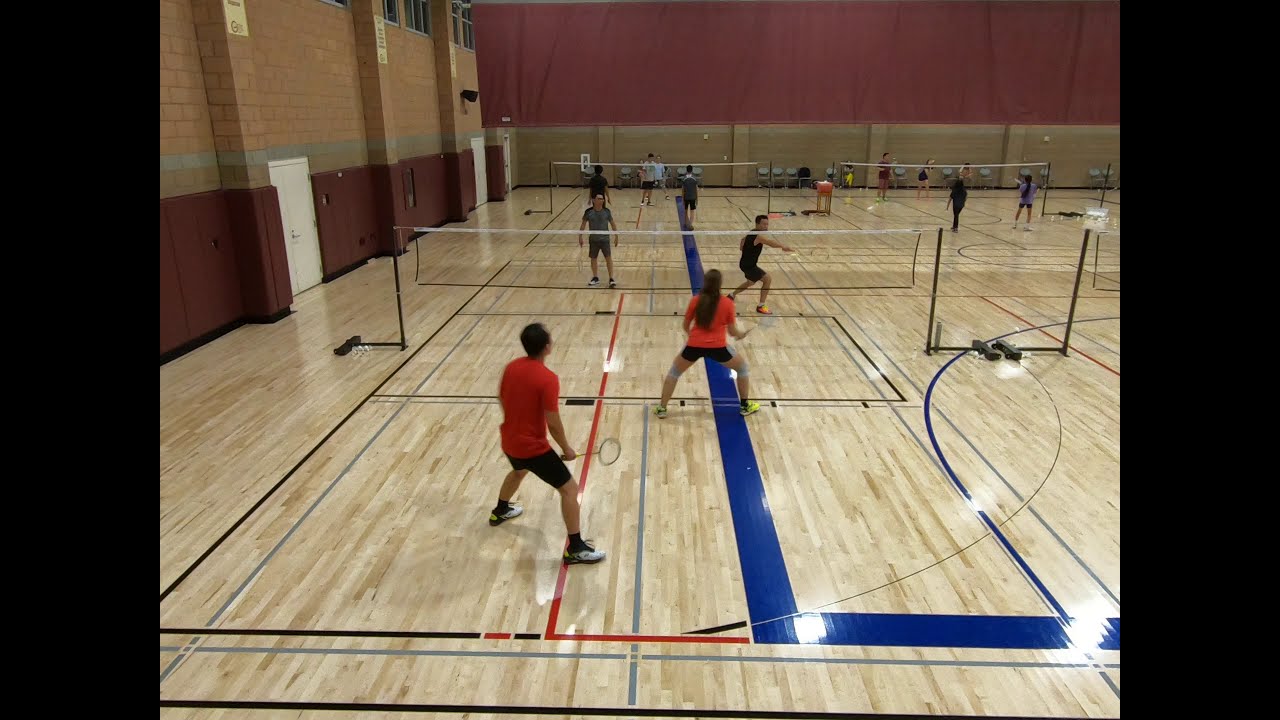The image depicts an indoor sports complex set up for multiple games of badminton. The gym features wooden floors with lines demarcating the courts and three visible nets, suggesting at least three games in progress, possibly a fourth in the far right corner. The players, equipped with rackets, are engaged in doubles matches, with the main game in the foreground showing two men playing against a mixed pair. The gym's left wall is adorned with red padding at the bottom, transitioning to orange brick above, while the back wall displays folded bleachers with a large red cloth hanging along its length. The ceiling is notably high, and the atmosphere is busy yet organized, with players wearing athletic gear in various colors including red, black, and white. The overall ambiance suggests a recreational hour where individuals come to enjoy an athletic game of badminton.